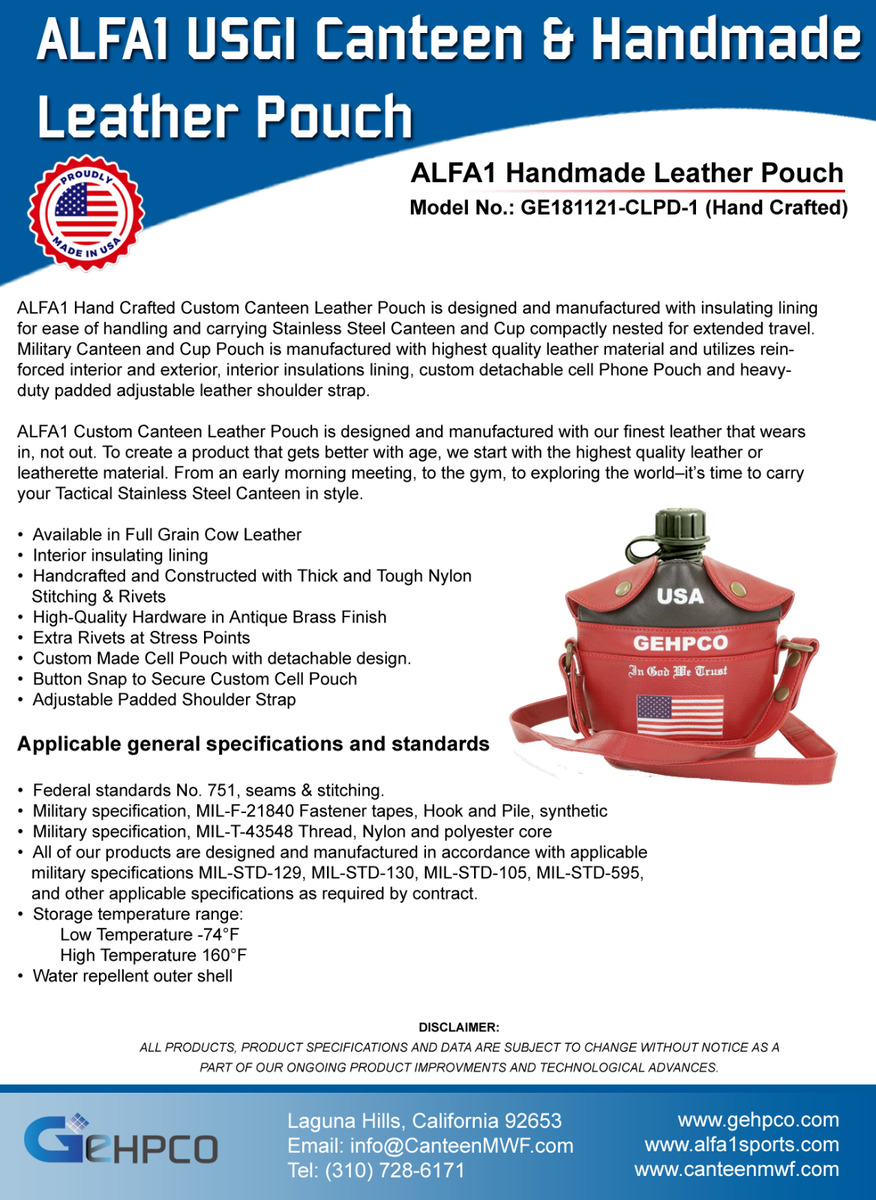This is a detailed advertisement for the ALFA1 USGI Canteen and Handmade Leather Pouch by Geph Gepco, prominently highlighting its quality and craftsmanship. At the top of the poster, in bold white capital letters, it reads "ALFA1 USGI Canteen and Handmade Leather Pouch." Adjacent to a red symbol and an emblem declaring the product "Proudly Made in the USA" is an image on the right side of the advertisement. The canteen itself is green, featuring a screw-on lid, and is nestled in a slightly reddish-brown leather pouch. This pouch is printed with "G.E.H.P.C.O." across it, accompanied by the inscription "In God We Trust" in white script above an American flag. The left side of the advertisement includes a list of features and specifications presented in bullet points under the heading "Applicable General Specifications and Standards." At the bottom, a notable footer with a blue bar contains the company address, contact information, and various websites, reinforcing the Geph Gepco brand's identity.